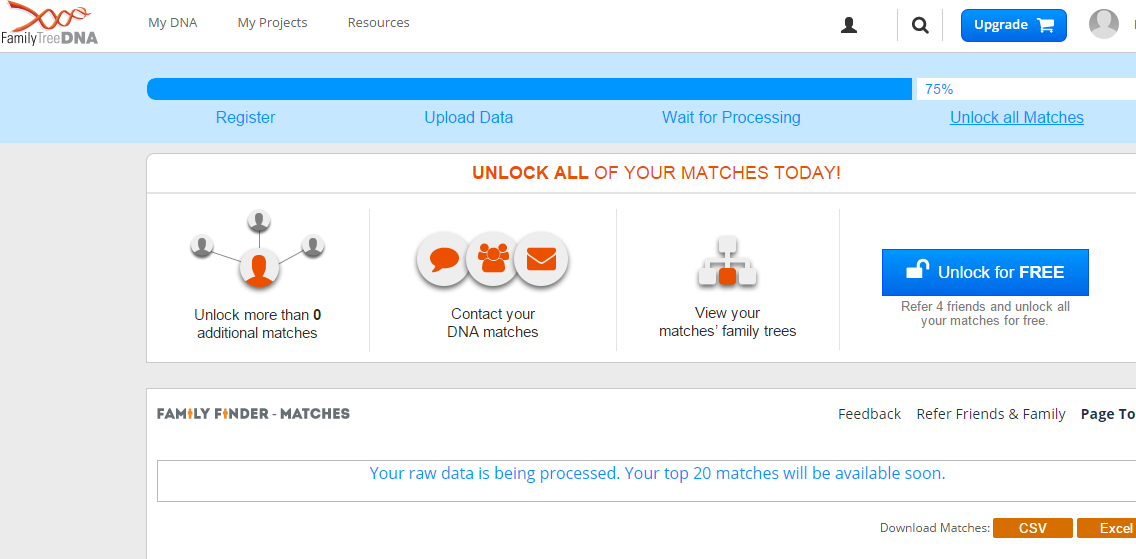This image is a screenshot of the Family Tree DNA website in landscape mode. In the upper left-hand corner, there is the Family Tree DNA logo, featuring an orange ribbon resembling a DNA strand winding in and out. Adjacent to the logo, at the top of the page, are four options: "My DNA," "My Projects," "Resources," and "Help." 

On the upper right-hand corner of the page, there is a person icon, a search icon, a blue button labeled "Upgrade" with a shopping cart icon, and a grayed-out avatar.

Below the navigation bar, there is a light blue background housing a progress bar that shows 75% completion, highlighted in blue with a white backdrop. Listed below the progress bar are several milestones: "Register" (marked as done), "Upload Data" (marked as done), and "Wait for Processing" (marked as done). The current status is "Unlock All Matches," underlined and in blue, indicating it's at 75%.

The main section is divided into two columns. On the left, there is a red heading stating "Unlock All of Your Matches Today." Below this, it offers the benefits of unlocking more matches, contacting DNA matches, and viewing their family trees. On the right, there's a button featuring an unlock icon that reads "Unlock for Free." Additionally, it mentions that you can refer friends to unlock all your matches for free.

Subsequently, there's a section titled "Family Finder Matches." To the right, details such as "Feedback," "Refer Friends," and "Your Raw Data is Being Processed" are outlined, stating that "Your top 20 matches will be available soon." At the bottom right of this section, there are two orange buttons labeled "CSV" and "Excel," which allow users to download their matches.